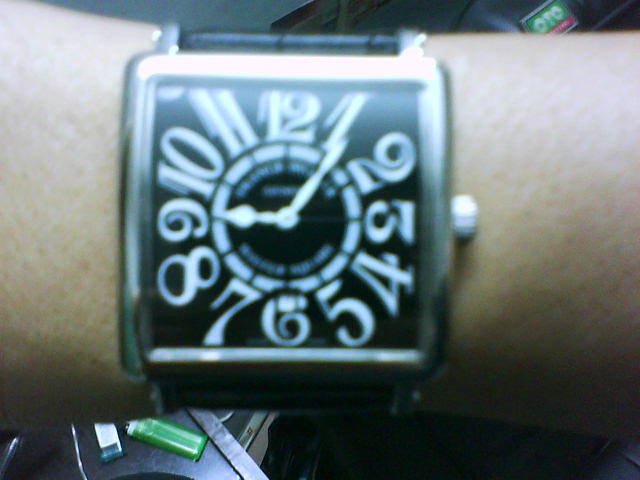The photograph centers on a wristwatch prominently displayed on a person's tan-colored arm, which is otherwise nondescript. The wristwatch itself is the focal point of the image, characterized by its distinctive silver metal square bezel enclosing a black face. The watch's dial features white, calligraphy-styled numerals ranging from 1 to 12, offering a unique aesthetic touch. Surrounding these numerals are white hash marks that form a precise circle. The watch's hands are also white, indicating the time as 9:06.

In the background, muted hues of brown and gray can be seen, providing a neutral backdrop that emphasizes the wristwatch. A green lighter is visibly placed within this background, adding a subtle, contrasting detail to the overall composition.